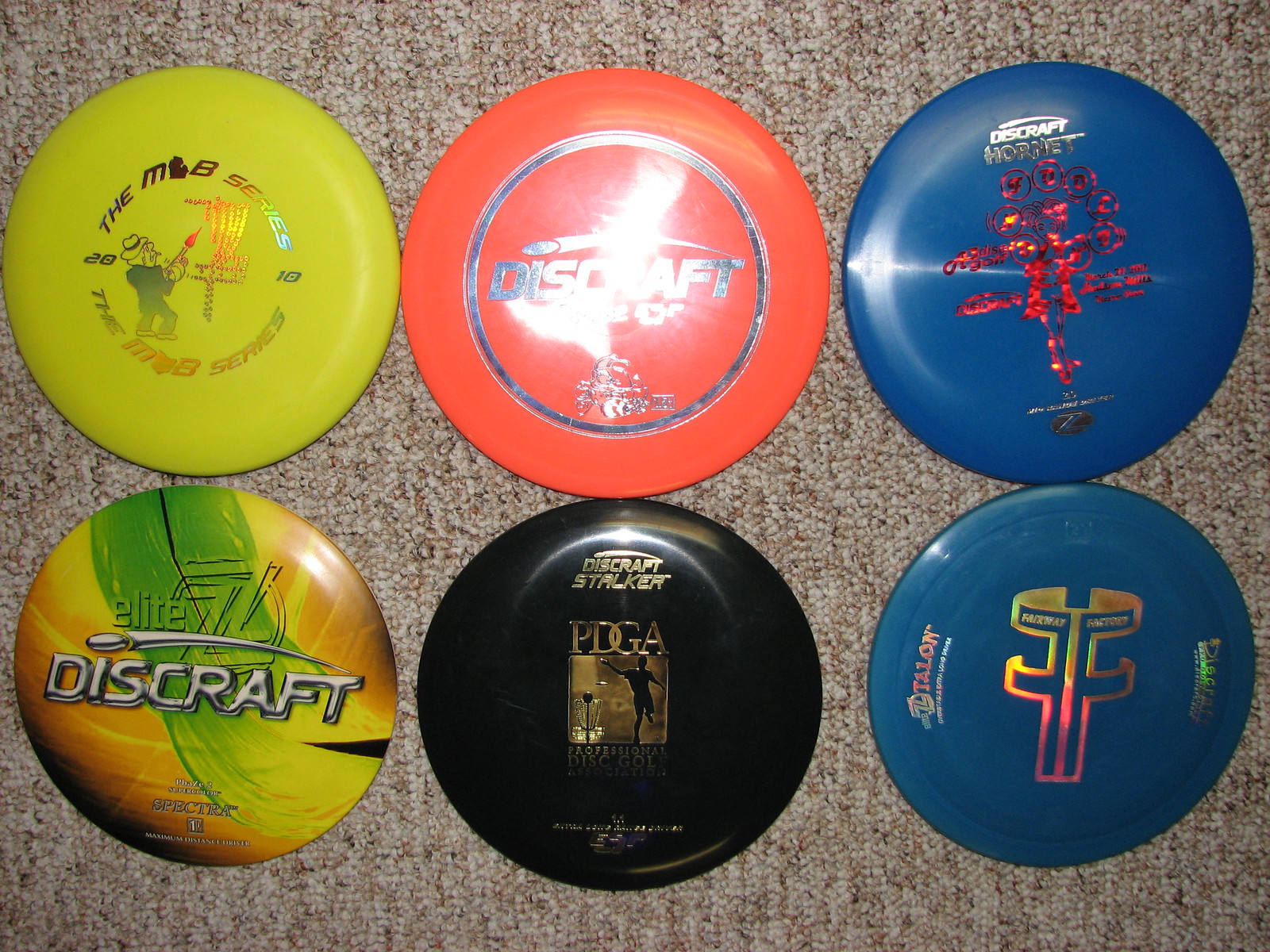This photograph showcases six well-worn disc golf frisbees arranged on a tightly-woven, brownish-red carpet akin to those found in hotel rooms or apartment buildings. Each frisbee features distinct colors and logos:

1. **Top Left**: A yellow frisbee labelled "The MB Series," showcasing a small character seemingly in action.
2. **Top Middle**: An orange and silver Discraft frisbee, though some text is difficult to decipher.
3. **Top Right**: A blue Discraft frisbee with a red design, also featuring partially illegible text.
4. **Bottom Left**: A green, orange, and yellow Discraft Elite Z frisbee.
5. **Bottom Middle**: A black Disc Golf frisbee with a gold PDGA (Professional Disc Golf Association) logo.
6. **Bottom Right**: A blue frisbee adorned with a gold and purple design and more text that is hard to read.

The frisbees look heavily used, but are neatly laid out for display, with each featuring various intricate logos and characters relevant to the sport of disc golf.